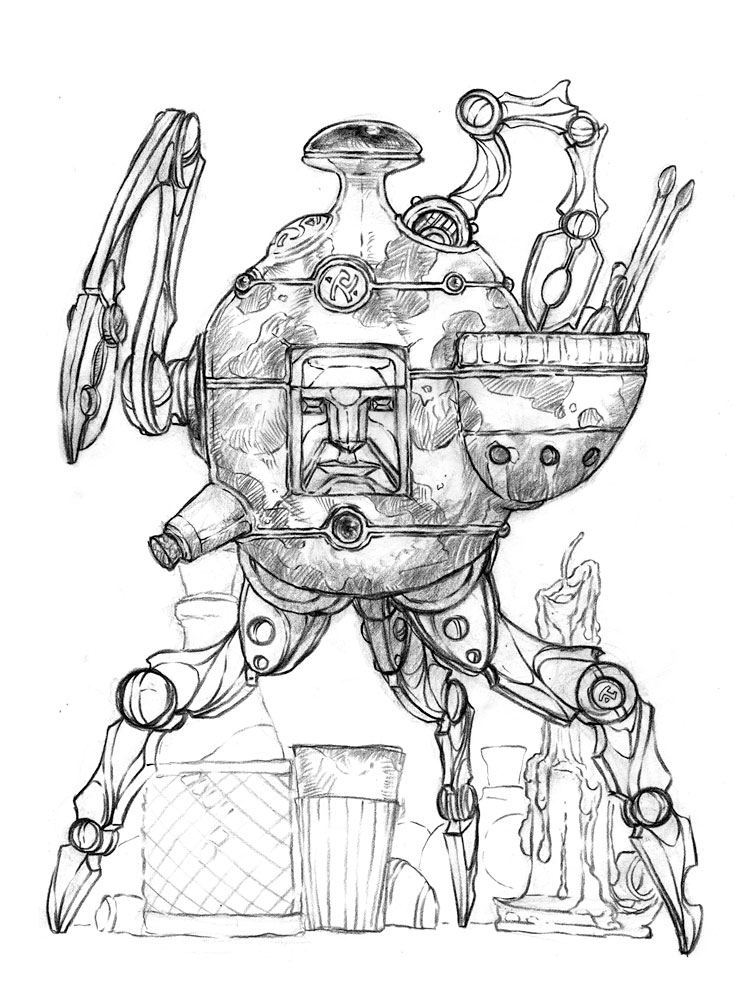The image is a detailed, pencil-drawn picture of a small-scale robot set against a white background. The robot, reminiscent of a metal contraption, features a round, bottle-like body adorned with various knobs and bumps. On the front of its body is etched a square-like humanoid face. It stands on three pointed, jointed legs resembling those of a tripod, each with two pivot points akin to knees and ankles.

One of the robot's arms, clawed like a lobster's pincers, extends from a knob on the left side of its body. Another identical arm extends downward from the very top of the robot toward a built-in basket on its right side, which contains various tools such as brushes and another knob. The top of the robot is finished with a circular dome.

In the background, everyday items like a bottle, a cup, and a melted candle provide context for the robot's diminutive size and suggest that it is standing on a kitchen counter-like surface.